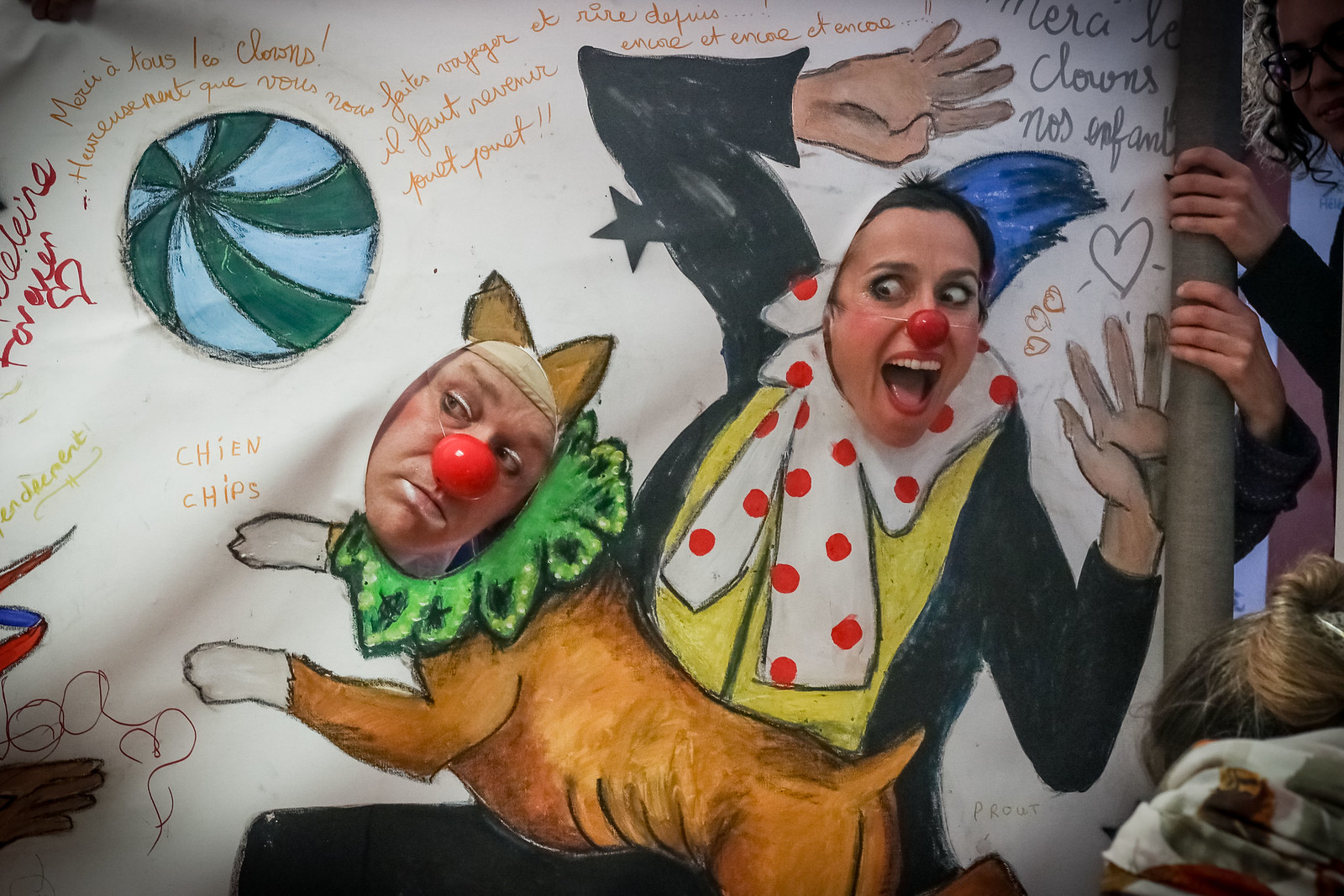The image features a humorous and whimsical scene set against a background with various colorful texts and abstract art, one of which reads "Chien and Chips." In the picture, there are painted character cutouts in a panel with holes where their heads should be, allowing people to poke their heads through. On the left, a man has his head through the cutout of a dog, which has a gray neckwear. The man, who has a big red clown nose, sports a sly expression as he looks upwards. On the right, a woman has her head through the cutout of a clown. The clown character has blue hair, a white neckpiece with red polka dots, and a yellow shirt. The woman, also wearing a big red clown nose, has her mouth wide open and eyes exaggeratedly wide, adding to the comic effect. The characters are depicted with their arms raised in a playful manner. An onlooker is visible on the side, observing the amusing scene as it unfolds, suggesting the photo was taken at a fun event such as a carnival or circus.